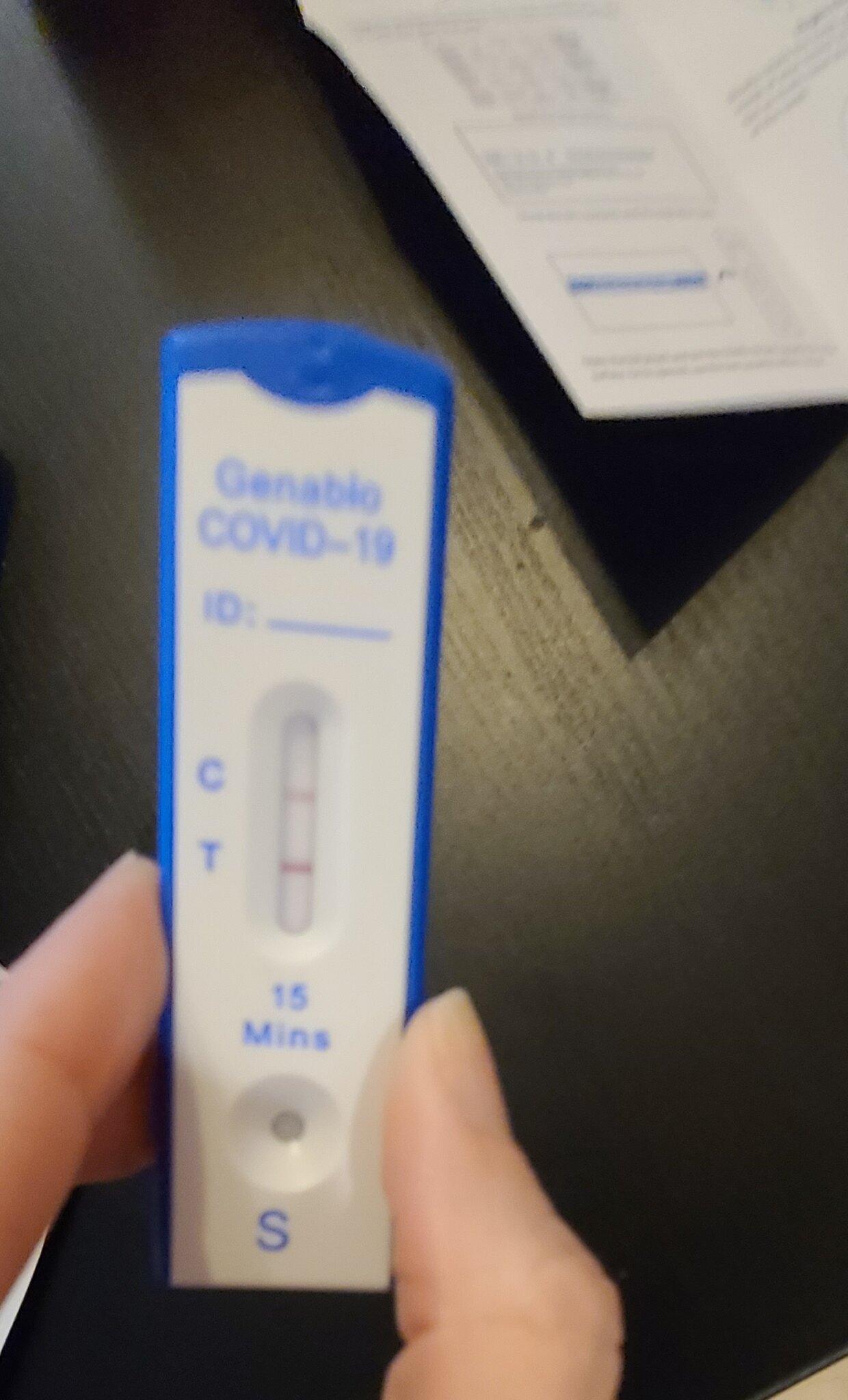In this detailed image, a person's fingers are prominently holding up a COVID-19 test kit made of plastic. The test is rectangular and features a blue outer edge with a white interior. Blue lettering on the test states "Generic COVID-19" at the top. Below that, there's an area labeled "ID:" followed by an underline space. Beneath this text is a small, clear meter that runs vertically. To the left of the meter, the letters "C" and "T" are positioned sequentially, with "C" at the top and "T" below it. Just under the meter, the text reads "15 minutes" in blue. The meter itself showcases two faint, light red lines in its center. Under the 15-minute mark is a small circle containing a dot, labeled with the letter "S." The fingers of the hand holding the test—thumb, index, and middle finger—are clearly visible. In the background, a dark brown table and a white pamphlet or book can be seen. The pamphlet, likely the instruction packet for the test, is positioned in the top right-hand corner of the image, placed on the table.